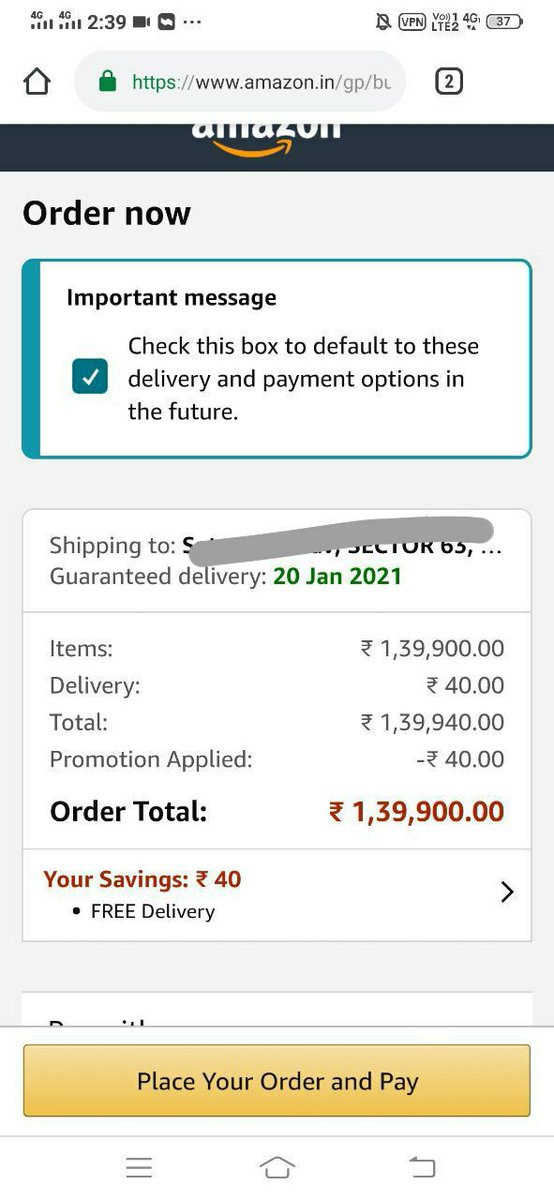A screenshot captures an Amazon order page, suggesting a very high-value purchase. The timestamp indicates it's 2:39, likely PM, though the location and exact time zone are unspecified. Wi-Fi is being used for the internet connection, and the device's battery is about half charged. The browser shows two tabs open, and it appears the user is screen recording their activity.

The order section prominently displays a message: "Important message: check this box to default to these delivery and payment options in the future," but the user evidently chose not to use the same payment method again. The shipping address has been redacted for privacy, with a guaranteed delivery date set for January 20th, 2021, highlighting the screenshot's age.

The item subtotal is an exorbitant figure, amounting to approximately a million units of an unspecified currency. Shipping costs are listed at $40, but a promotional discount of $40 is applied, resulting in a net free delivery. The total cost and final price, including the discount, are clearly shown just above the "Place your order and pay" button at the bottom of the page.